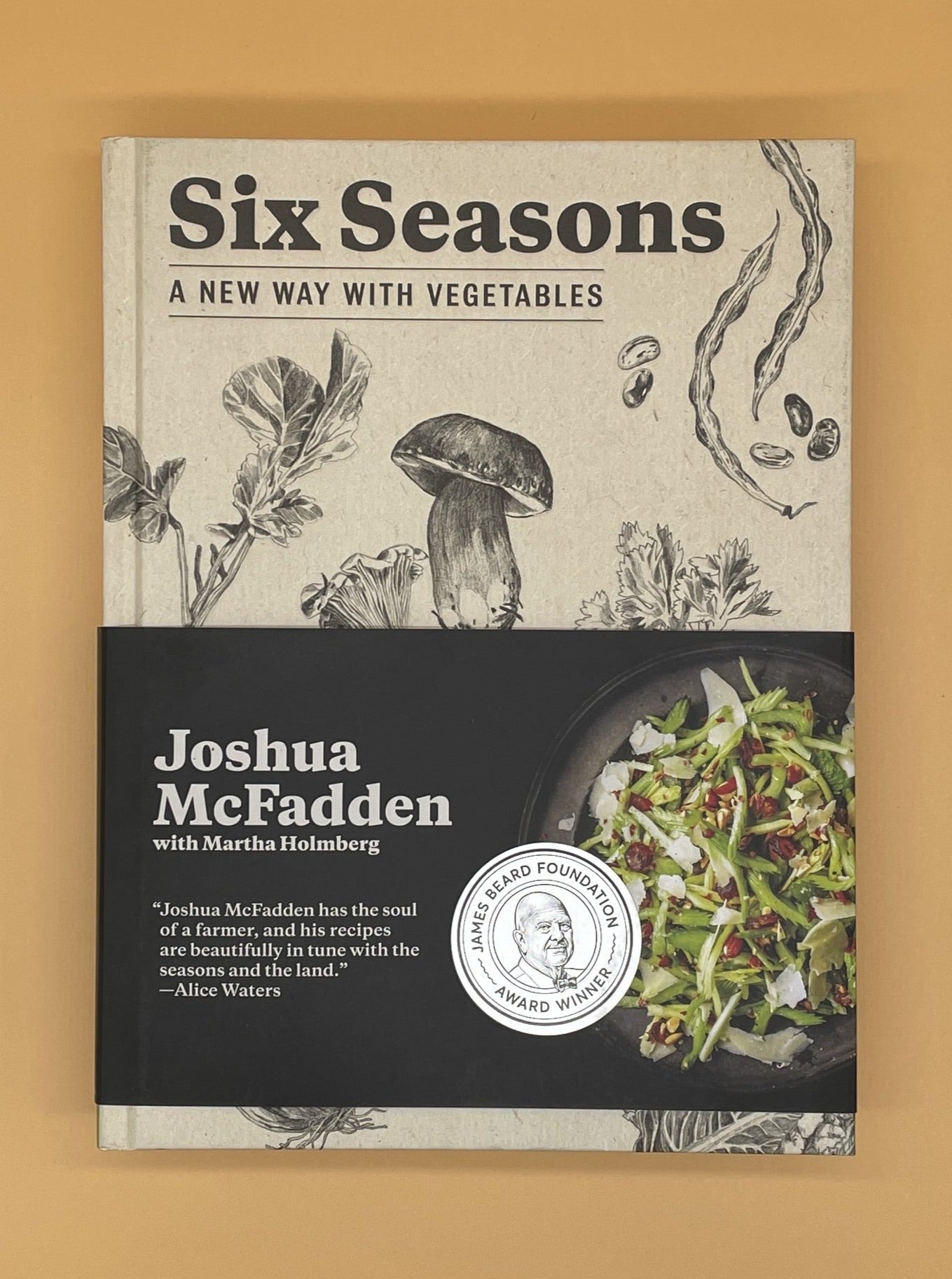This photograph captures the book "Six Seasons: A New Way with Vegetables" by Joshua McFadden with Martha Holmberg, prominently placed on a nondescript table. The cover features a minimalistic, off-white background with bold black typography. The top half of the cover showcases a striking black-and-white image of a mushroom, accented with beans and green foliage, emphasizing the book's focus on seasonal vegetables. Below this, a black banner stretches across the cover, displaying a tantalizing photograph of a vibrant, unconventional salad, hinting at the innovative recipes within. The endorsement from Alice Waters praises McFadden's deep understanding of the land and seasonal produce, reading, "Joshua McFadden has the soul of a farmer, and his recipes are beautifully in tune with the seasons and the land." This critical acclaim, coupled with the James Beard Foundation Award seal, attests to the book's distinguished reputation in the culinary world.